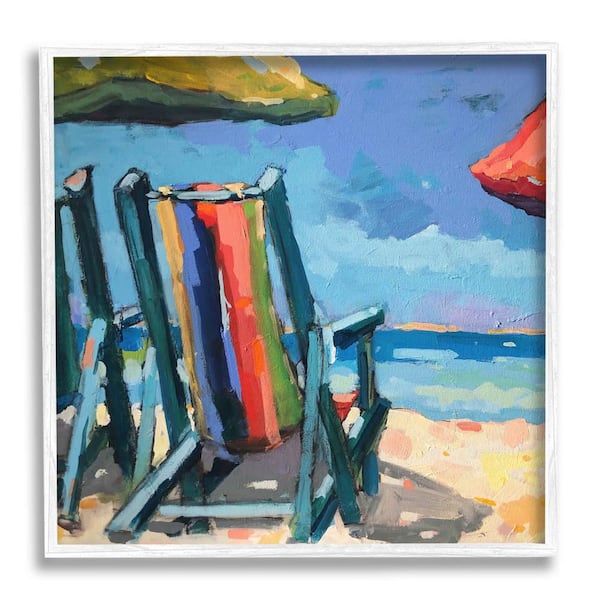This vibrant oil painting portrays a serene beach scene featuring two empty beach chairs resting on a sandy shore. The sand is depicted with a warm palette of tan, yellow, orange, pink, and red hues. The chairs, with their blue frames, are distinguished by their colorful, vertically-striped fabric backs featuring alternating stripes of yellow, blue, pink, and green. On the left side, one chair is partially cut off. Overhead, a yellow umbrella provides shade, while a glimpse of a cut-off red umbrella appears on the right. The ocean stretches out into the distance, with darker blue hues in the background transitioning to lighter blue mixed with white nearer the shore, capturing the ebb and flow of the waves. The sky above is depicted as a cloudy day, with dark blue at the top and lighter blue with white clouds towards the horizon. In the background, subtle landforms add depth to the tranquil seascape. The painting is bordered by a white frame, though no artist's signature is visible.